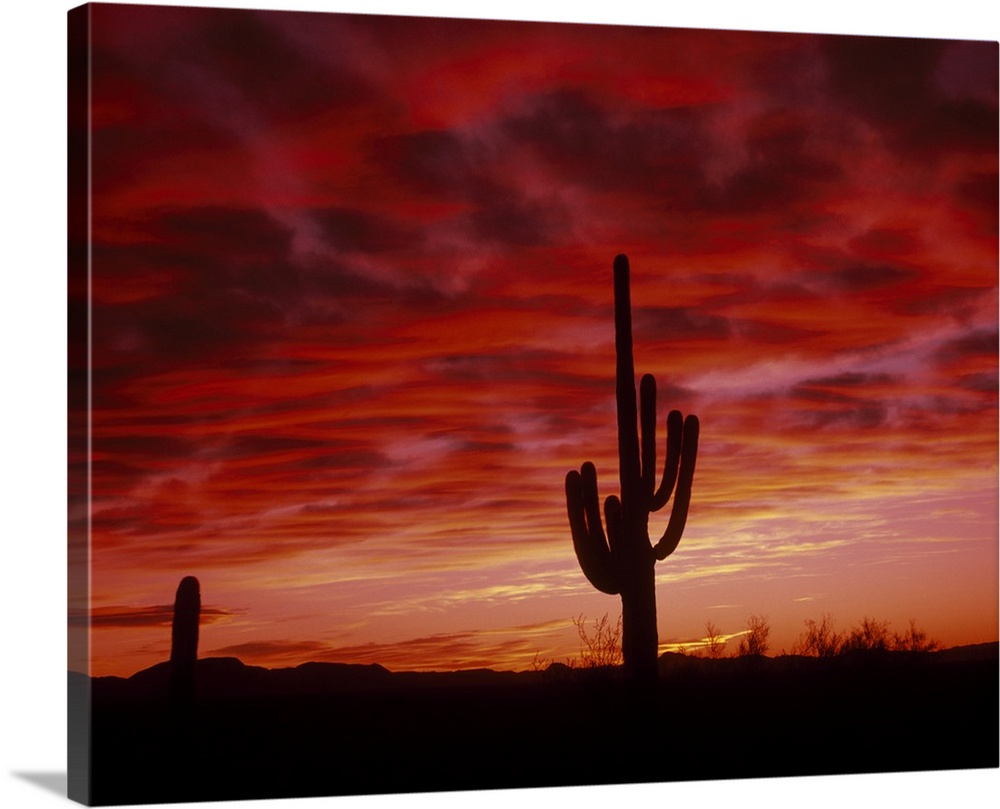The image features a digital render of a desert landscape, likely inspired by the Arizona desert, captured at dusk. It presents a vivid evening sky ablaze with vibrant hues of deep red, pink, gold, yellow, and purple, giving the impression that the sky is on fire. The primary focus is on two silhouetted cacti, with one prominently standing tall while the other is positioned off to the side. These cacti are rendered in black, emphasizing their shadowed forms against the colorful backdrop. Puffy clouds are scattered across the sky, and distant mountains and shrubs further evoke the desert setting. The image is depicted on a 3D-rendered block, intended to resemble a canvas hanging at an angle, adding a sense of depth and dimension to the scene.